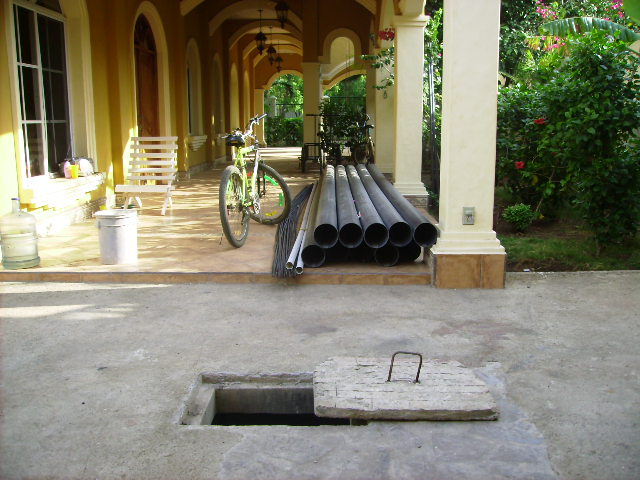The image depicts a detailed scene of a grand, old house, likely built a century or two ago, featuring Spanish architecture with an expansive veranda at the forefront. The veranda is adorned with an arched roof supported by pillars, and a variety of items are scattered around: a parked bicycle, white chairs, metal pipes of various sizes, cables, and buckets. The veranda seamlessly merges into a cement path, which occupies the lower half of the image. Prominently on the path is a rectangular manhole cover, made from a light-colored material like beige metal or cement, which has been removed to reveal a hole beneath. On the right side of the veranda area, lush greenery can be seen, including shrubs, possibly a rose bush, and potentially a leaf from a banana tree, indicating a rich garden surrounding the house.